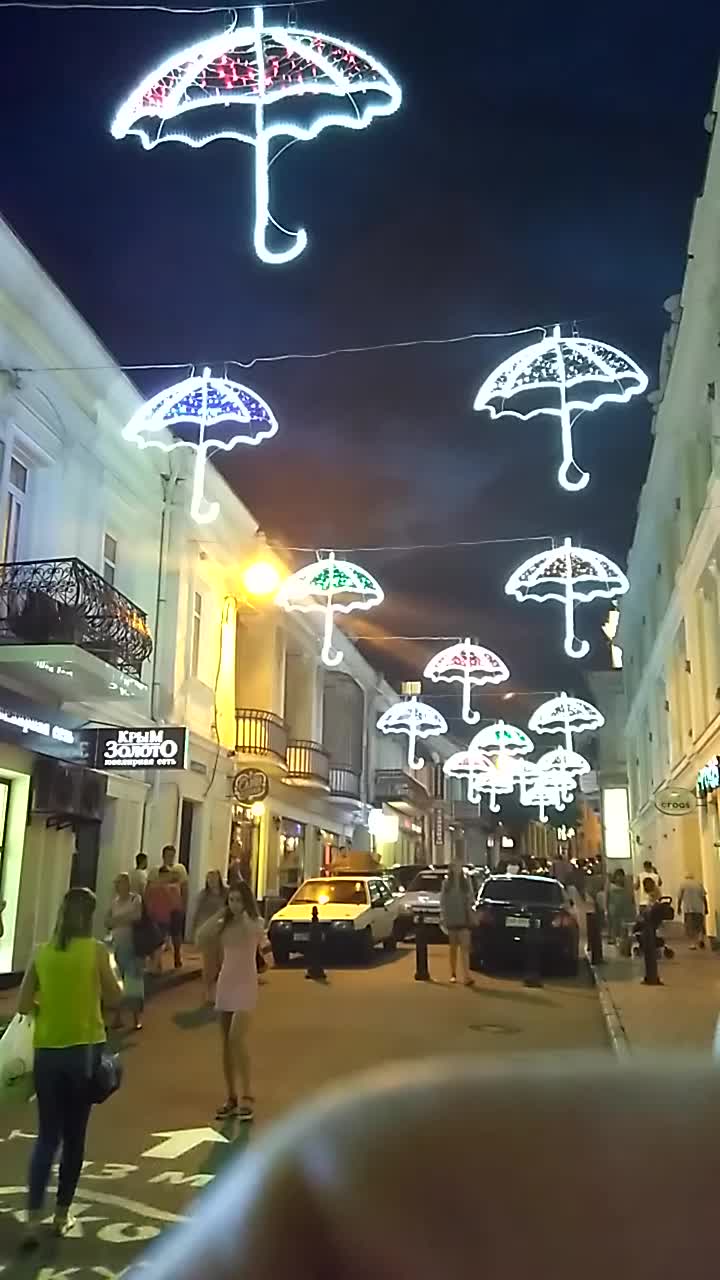The photograph captures a bustling, narrow alleyway between elegant white apartment buildings adorned with balconies. It's nighttime, lending a whimsical glow to the scene illuminated by an array of lighted umbrellas that stretch across the street on multiple wires, creating a mesmerizing canopy of neon colors—blue, red, green, and white. This alley, likely a shopping district in a foreign country as suggested by the signage in a different language, is lively and chaotic with people walking down the street and on the sidewalks, some taking photos of one another. Despite the nighttime setting, the street is vibrant with activity, including a mother capturing a picture of her daughter against the backdrop of glowing umbrellas. Cars are parked haphazardly, accentuating the narrowness of the street, but restricted from entering past a certain point by barriers. Neon signs further brighten the scene, providing a picturesque travel destination that suggests a pleasant night out for both locals and tourists.